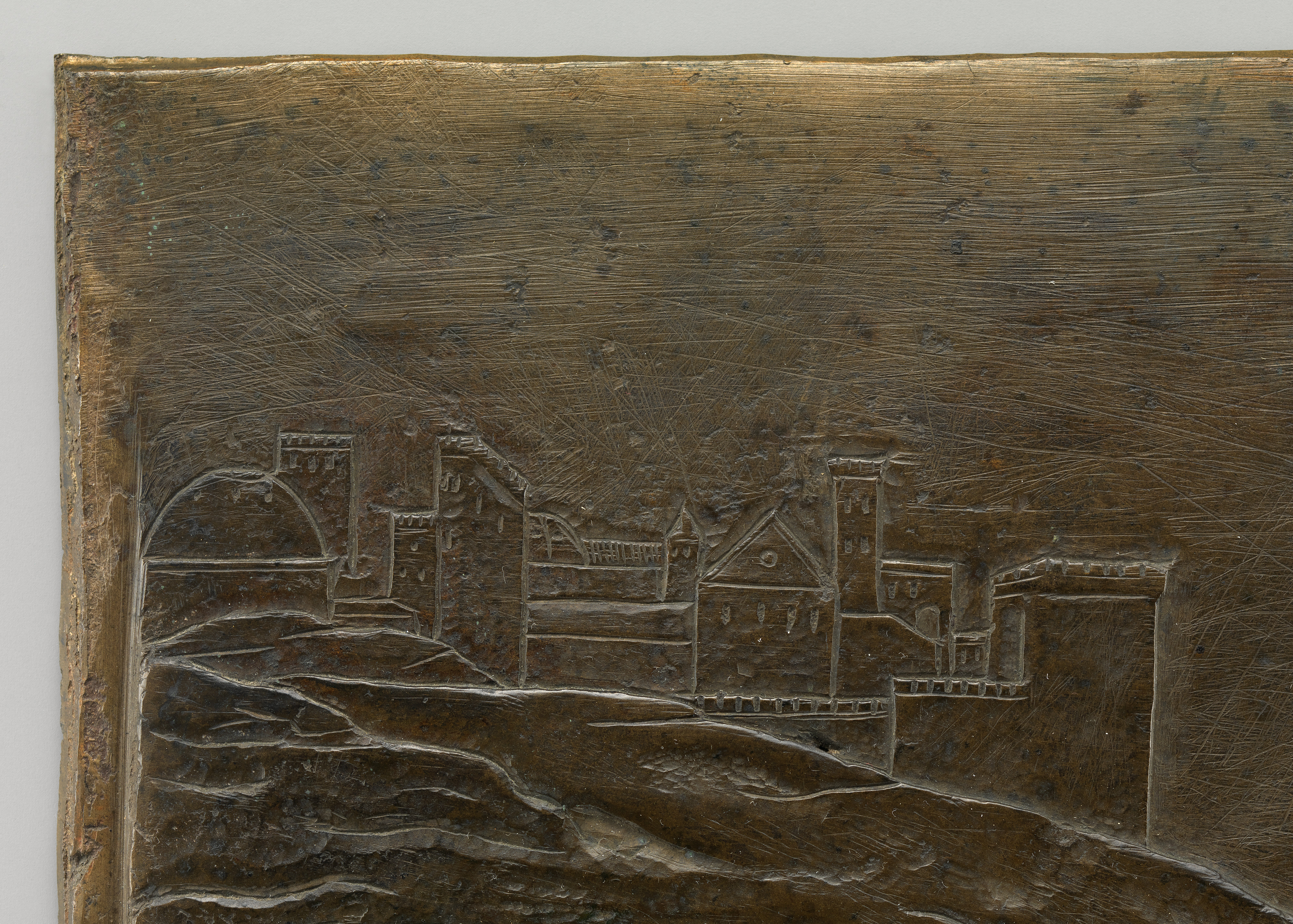This detailed image depicts a carved wooden artwork mounted against a gray background, possibly displayed in an art gallery. The central focus is a cityscape illustrated through simplistic carved lines on gold-toned brown wood. A golden sheen, enhanced by overhead lighting, highlights the horizontal striations traversing the wood's surface. 

In the foreground, a carved hillside slopes from the center left downward to the bottom right, appearing rocky and textured. The city buildings etched into the wood above this hillside are characterized by their minimalist design, using basic shapes like squares and lines. 

Prominently, the city features a round building with a domed roof on the left. Behind it stands a square tower with three windows, juxtaposed with a rectangular tower and a sloped roof in the foreground. Further back, a distinct building resembling a church with a steeple and clock stands, alongside another structure with an A-frame roof, possibly hinting at a government building. The background, representing the sky, is left largely uncarved, showcasing flowing brown tones punctuated by scratches, enhancing the rustic and crafted aesthetics of this captivating wooden artwork.